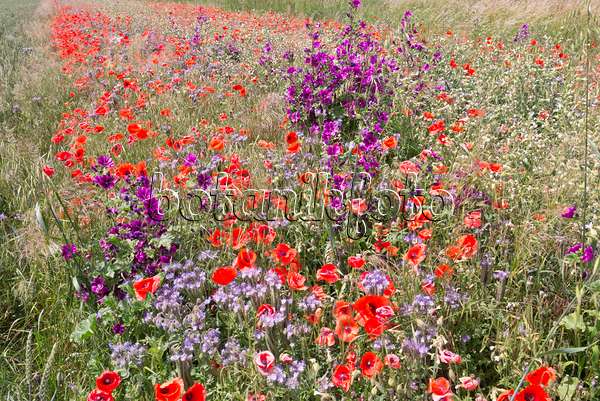The image depicts a field of wildflowers with hues of light purple, dark purple, red, and woven green vegetation basking in the daylight, though the sun itself is not visible. The colors in the scene are pastel and muted, contributing to a serene ambiance. The lower-resolution photograph appears grainy, and any fine details in the flowers or grass are subdued. Spanning across the center is a watermark with a raised, scrawly typeset that reads "B-O-T-A-N-I-K-F-O-T-O," which blends semi-translucently into the floral background. The image and the watermark suggest an unprofessionally done logo or one that has been excessively enlarged, hence the pixelation. The field of flowers extends into the distance, enhancing the image's sense of depth despite its graininess.